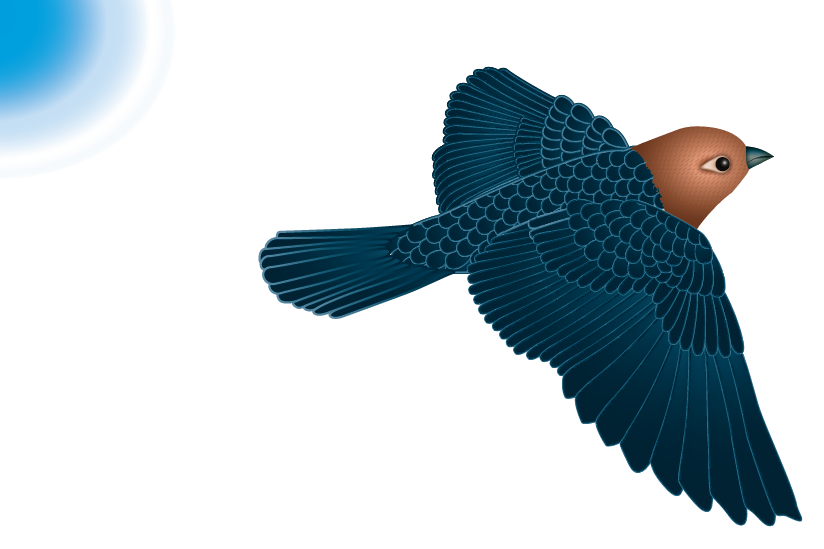This detailed illustration depicts a stylized bird flying against a stark white background. In the top left corner, there is a blue orb resembling a quarter-sun, emanating subtle gray and white stripes. The bird is positioned centrally, flying towards the right with wings outstretched. The bird's head has a rich brown color, featuring a distinct black beak with hints of greenish-blue, and a prominent black pupil with a white and yellow-tinged iris. The body and wings are dark royal blue with a unique pattern: the body and top side of the wings have a fish-scale-like texture, while the underside of the wings and the tail showcase more traditional feather features. The pattern extends throughout the bird, blending seamlessly to create an animated, yet intricate appearance. The entire image, devoid of any additional scenery, emphasizes the bird and the contrasting blue sun against the plain white sky.